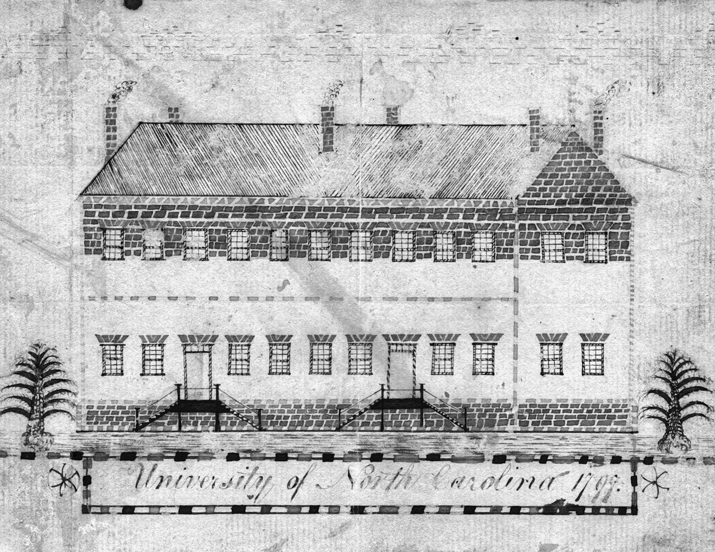This image is a black-and-white, pencil drawing that appears to be very old and weathered. It depicts a rectangular, two-story building with a slanted roof adorned with six chimneys, some emitting smoke. The building has distinct sections: a top section of brick siding with 12 windows, a middle white section with 10 more windows and two doors, and another brick section at the bottom with small porches and steps leading to each door. The background is gray, further adding to the aged appearance of the drawing. There are two trees flanking the building—one on each side—which appear shorter and somewhat resemble palm trees. At the bottom of the image is a sign reading "University of North Carolina, 1799," although the last two digits are slightly unclear, potentially reading '98 or '97. The overall impression is of an aged, detailed sketch of the historic university building.